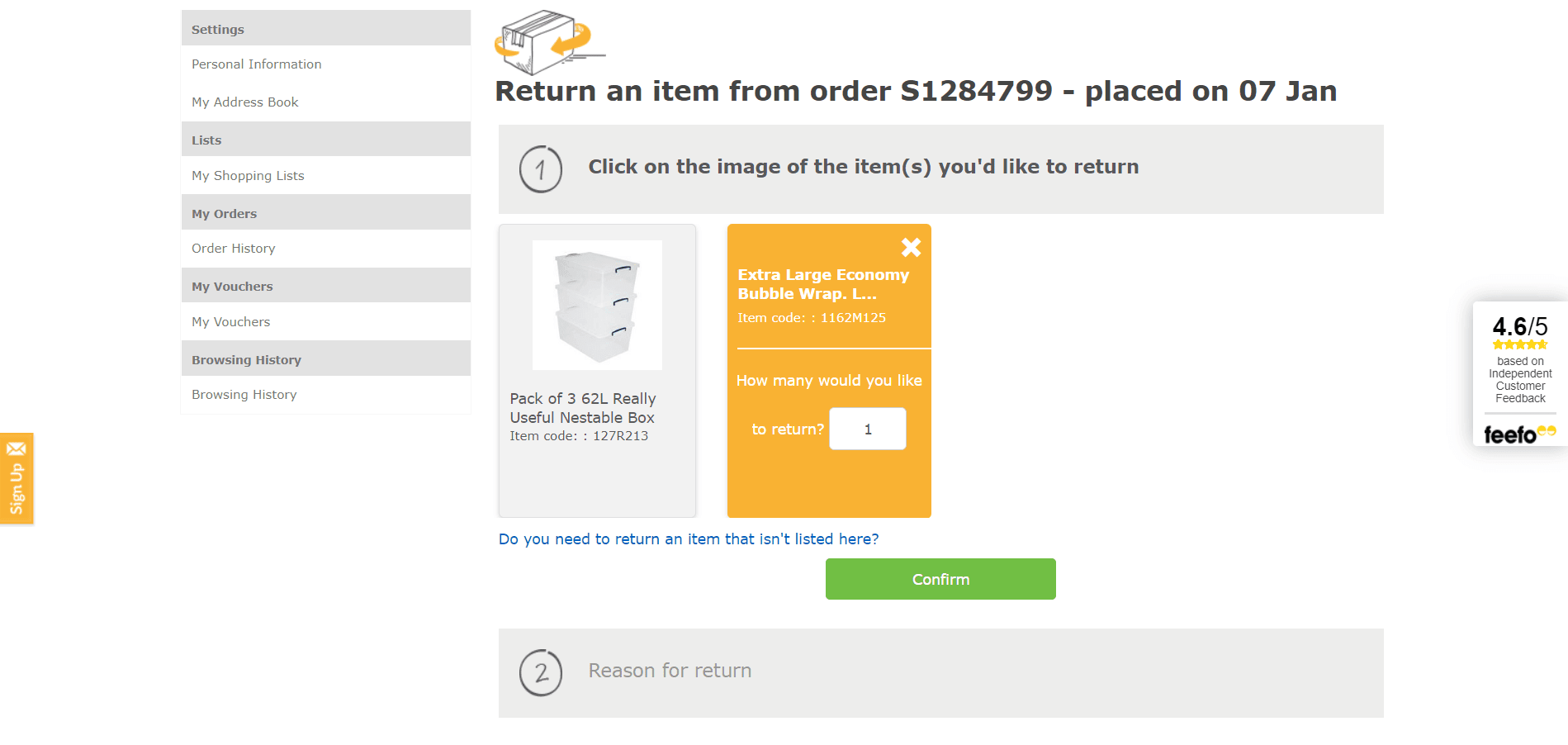This is a detailed screenshot of someone initiating a return for an item ordered from a website, likely named FIFO. On the right side of the screen, a small tag displays a rating of 4.6 out of 5 based on independent customer feedback, with the word "FIFO" prominently featured. Central to the image is the title "Return an item for order S-1284799 placed on 07 Jan" followed by a step-by-step guide.

Step 1 instructs the user to click on the image of the items they wish to return. Below this instruction are images of the items with captions. The first item is a "Pack of 362L Really Useful Nestable Boxes" accompanied by its item code. To the right, another product is labeled "Extra Large Economy-Level Wrap," also with its item code. A box beside this product allows the user to specify the quantity to return, currently showing the number 1.

Further down, a prompt asks "Do you need to return an item that isn't listed here?" followed by a green "Confirm" button. Below this button, a second step titled "Reason for return" is partially visible, indicating that the user has not scrolled down enough to view it fully.

On the left side of the screen, a vertical navigation bar lists various options: "Settings," "Personal Information and My Address Book," "Lists," "My Shopping List," "My Orders," "Order History," "My Vouchers," "Browsing History," and another identical set of "My Vouchers" and "Browsing History."

The overall color scheme of the webpage is primarily gray and white, accentuated by hints of orange, yellow, and green.